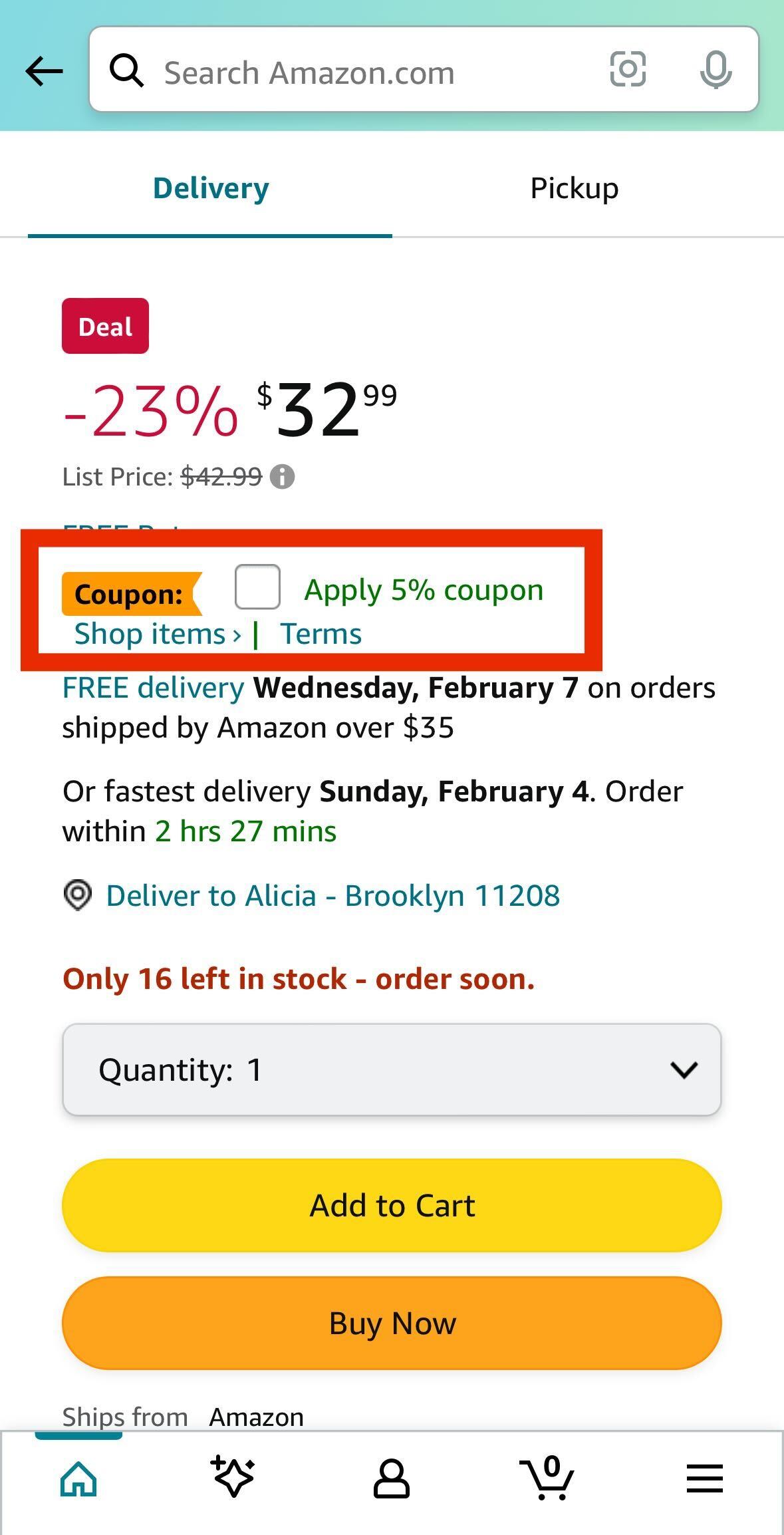**Detailed Caption:**

The image features an interface with a light blue border at the top. On the left side, there is an arrow pointing to the left. Immediately below, a search bar displays the text "searchamazon.com." 

Beneath the search bar, the section labeled "Delivery and Pickup" is displayed, with the word "Delivery" highlighted in blue and underlined. Directly below, a red box labeled "Deal" is shown, followed by text in red that indicates "-23%". The current price is listed in black as "$32.99," with the original list price noted as "$42.99."

Additionally, there is an orange or red rectangular box highlighting an area that includes an orange ribbon with the word "Coupon." Inside this area, there is an empty checkbox adjacent to the text "Apply a 5% coupon." The words "Shop items and terms" are also present within this highlighted section.

Below the red box, delivery details are provided: "Free delivery Wednesday, February 7, on orders shipped by Amazon over $35, or fastest delivery Sunday, February 4. Deliver within 2 hours 27 minutes." Delivery is specified to be to "Alicia, Brooklyn 11208," with a quantity of "1."

At the bottom of the interface, there is a prominent yellow "Add to Cart" button next to an orange "Buy Now" button.